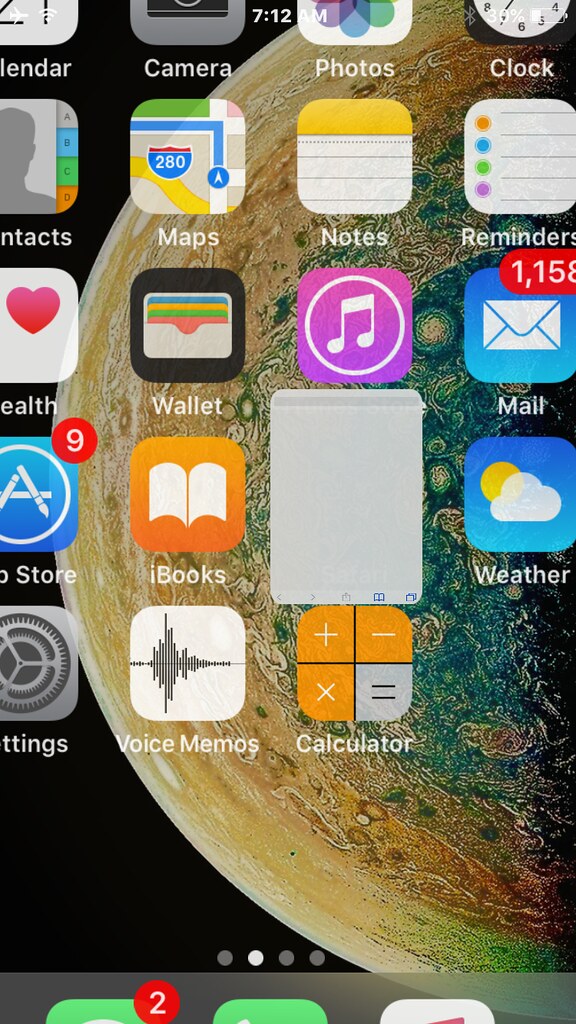A close-up view of a smartphone's home screen reveals a curious detail: a partial screenshot of what appears to be a search result is prominently displayed in the background, blending seamlessly with the actual screen. The image is zoomed in, obscuring the very top and bottom edges of the home screen, yet it captures an array of popularly used apps. From left to right, one can distinctly identify icons for Contacts, Maps, Notes, Reminders, Health, Wallet, and Music. Notably, the user's Mail app displays a staggering 1,158 unread messages, and the App Store icon shows nine pending updates.

A closer inspection reveals additional apps: Books, Weather, Settings, Voice Memos, and Calculator. Intriguingly, the screenshot superimposition lies immediately after the Books app icon. At the screen's bottom margin, partially cropped icons suggest the presence of the Messages and Phone apps, both denoted by green icons with unread notifications—though it’s difficult to determine which is which due to the zoomed perspective. Another unidentified white app with pink elements is also visible. 

Peeking from the top edge of the image are segments of the Calendar, Camera, Photos, and Clock apps. Indicators along the status bar divulge that the device is in Airplane Mode, connected to Wi-Fi, and currently 7:12 AM. The phone also has Bluetooth enabled and a remaining battery life of 30%.